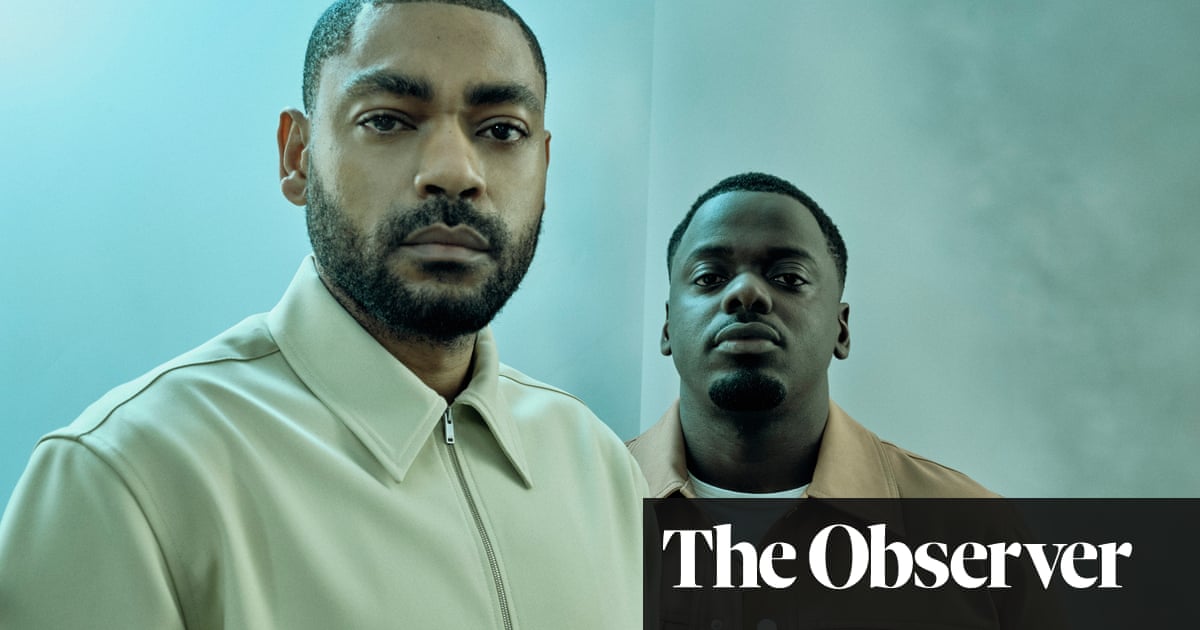This is a detailed photograph featured in The Observer, indicated by the black square logo with white print in the bottom right corner. The image has a bluish-green background and focuses on two young black men with slight variations in skin tone. The man on the left, who has a slightly lighter complexion, sports a light green collared shirt with a zipper down the front, complemented by a scruffy beard. He has a strong, determined expression on his face. The man on the right, likely actor Daniel Kaluuya from the film "Get Out," is dressed in a tan collared jacket over a white shirt. He has a calm demeanor, a close-cropped hairstyle, and a small goatee. Both men are looking directly at the camera, suggesting this may be part of a profile or advertisement within the publication.